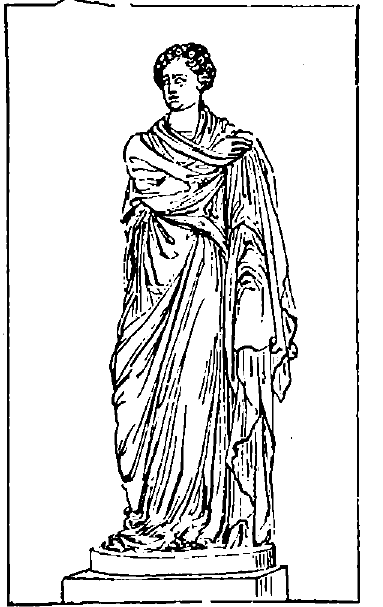The image is a black and white pen and ink drawing of an ancient statue, possibly depicting a Greek or Roman figure. The statue stands upright on a round plinth mounted atop a square base, set against a blank white background with a simple black line border that is slightly broken near the upper left corner. The figure is detailed with voluminous robes that drape intricately, creating numerous pleats and folds. The statue has short, curly hair and simplistic facial features, including eyes, a nose, and a mouth. The figure is facing the viewer but with its head tilted in a three-quarter profile, looking towards the left side of the image. The statue's right arm is raised to touch its left shoulder, while the left arm is draped down, obscured by the flowing garment. This portrayal provides a detailed, yet elegant glimpse into classical artistry, emphasizing the timeless grace of ancient statues.